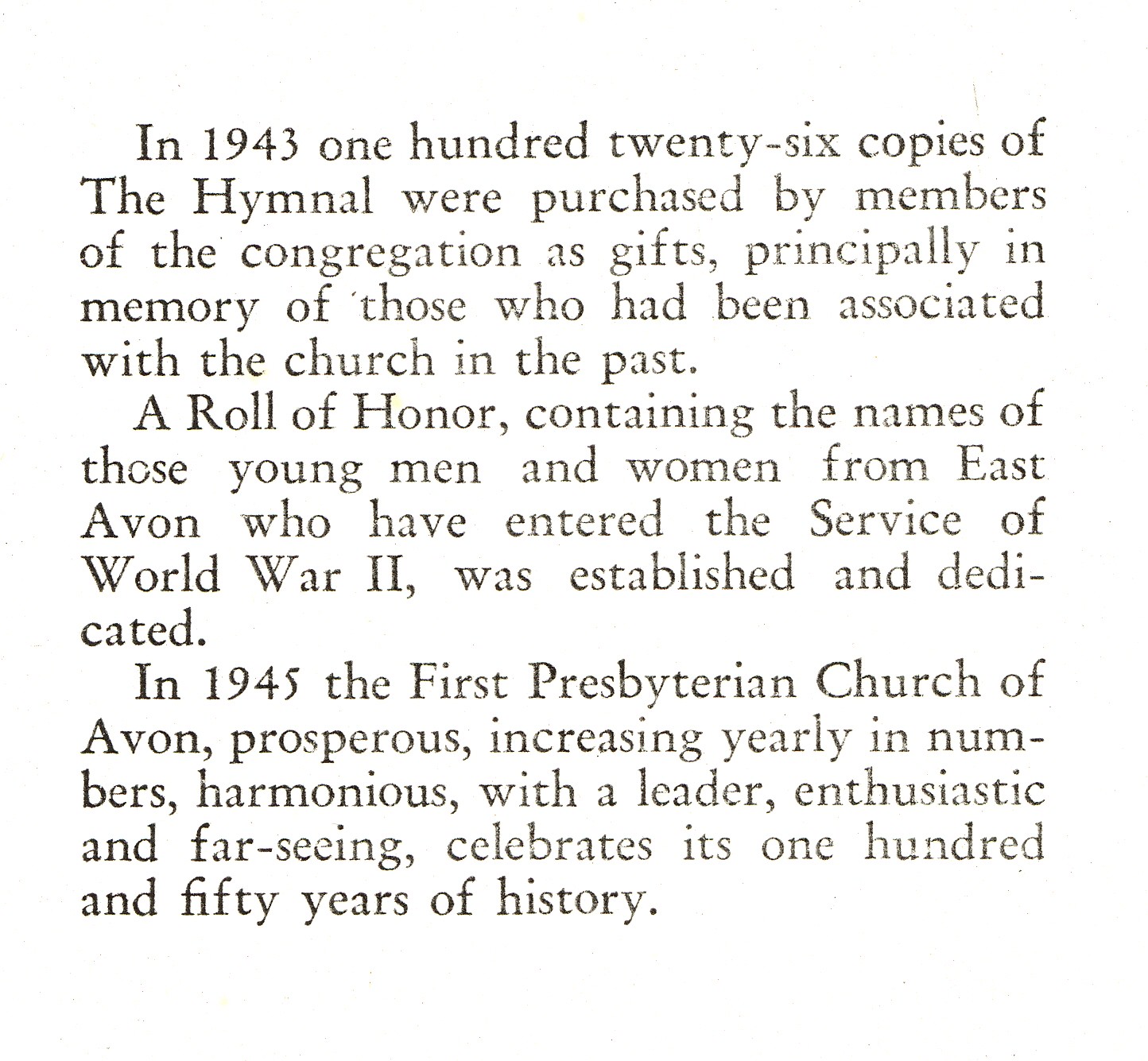The image is a scan likely from a book, magazine, or newspaper, featuring a completely white background with slightly choppy black text, indicating it is not an original but a photocopy or scan of a printed document. The black text is a bit grainy and faded. The text reads, "In 1943, 126 copies of the hymnal were purchased by members of the congregation as gifts, principally in memory of those who had been associated with the Church in the past. A roll of honor containing the names of those young men and women from East Avon who have entered the service of World War II was established and dedicated. In 1945, the First Presbyterian Church of Avon, prosperous, increasing yearly in numbers, harmonious with a leader, enthusiastic and foreseeing, celebrates its 150 years of history."